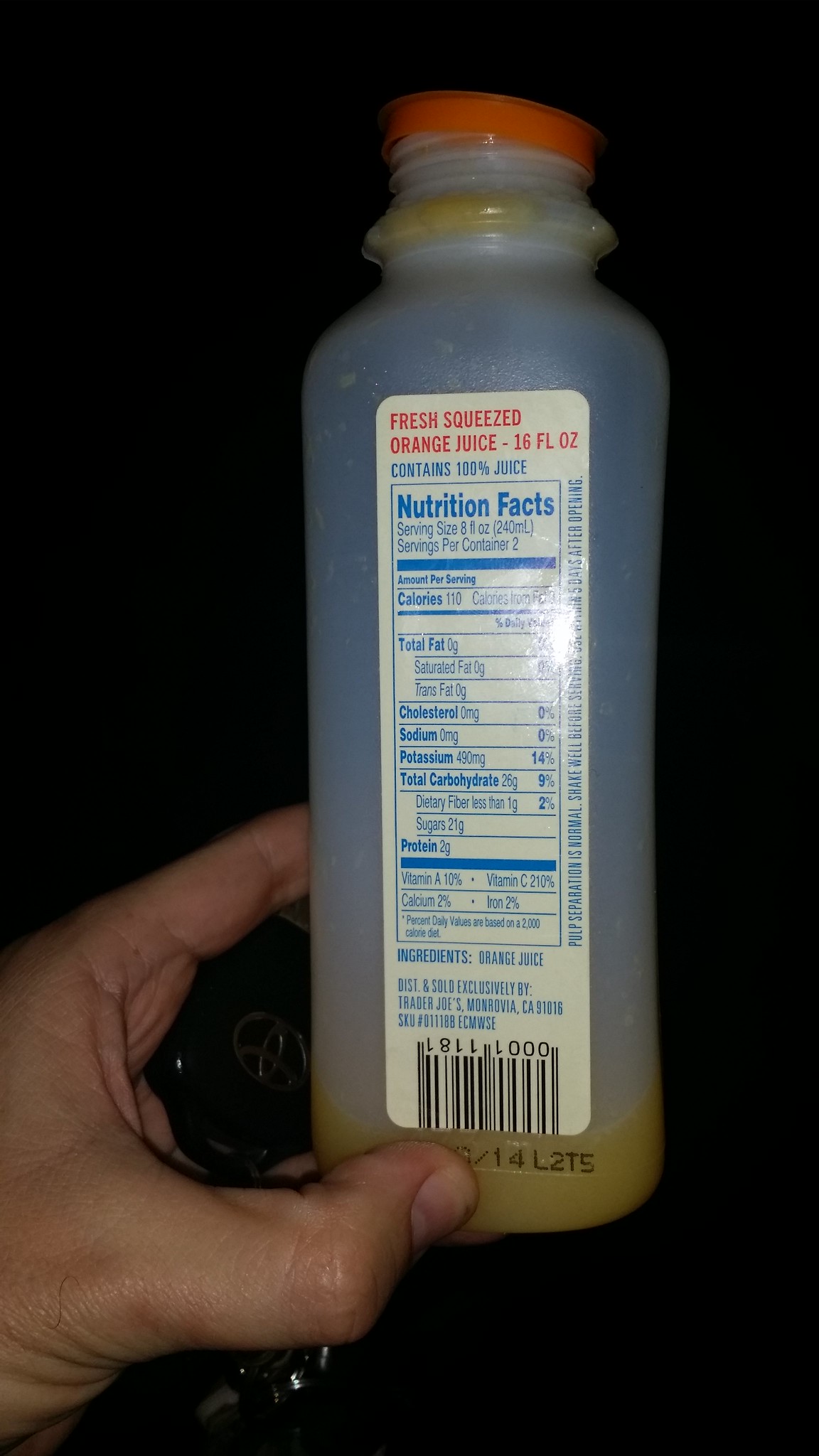A nearly empty, single-serving container of fresh-squeezed orange juice is held by a hand visible from the thumb up, coming in from the left side of a black background. The container, made of semi-opaque plastic, has only about a thumb’s worth of juice remaining at the bottom. The cap has been removed but rests on top of the container, revealing its orange color. The label reads "Fresh Squeezed Orange Juice, 16 Fluid Ounces" in red, and below, in blue, it states "Contains 100% Juice." Additionally, the nutrition facts on the label are visible, displaying 110 calories and information on total fat, cholesterol, sodium, potassium, and total carbohydrates. The only ingredient listed is orange juice.